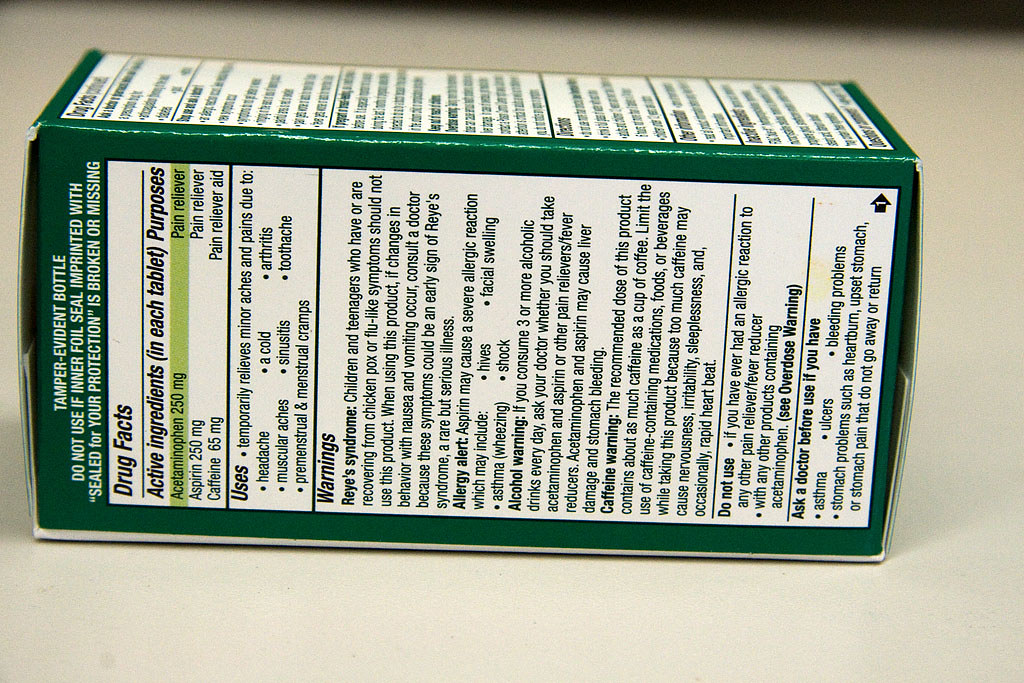This landscape-format color photograph depicts a medication box that has fallen onto its side on a flat white surface, making the text difficult to read without tilting your head to the left. The box shows the back side, featuring a green background with numerous warnings and drug information listed vertically. Key visible text includes, "Tamper evident bottle, do not use if inner foil seal imprinted with 'sealed for your protection' is broken or missing." It specifies drug facts, noting active ingredients such as acetaminophen (250 mg), aspirin (250 mg), and caffeine (65 mg), all of which are included for pain relief. Additional vertical text outlines uses for temporary relief of minor aches and pains from headaches, muscular aches, premenstrual and menstrual cramps, colds, sinus issues, arthritis, and toothaches. Numerous warnings are present, including about Reye's syndrome, allergies, alcohol, and caffeine. The top portion of the box, though blurry, contributes to the detailed presentation of the precautions and instructions.